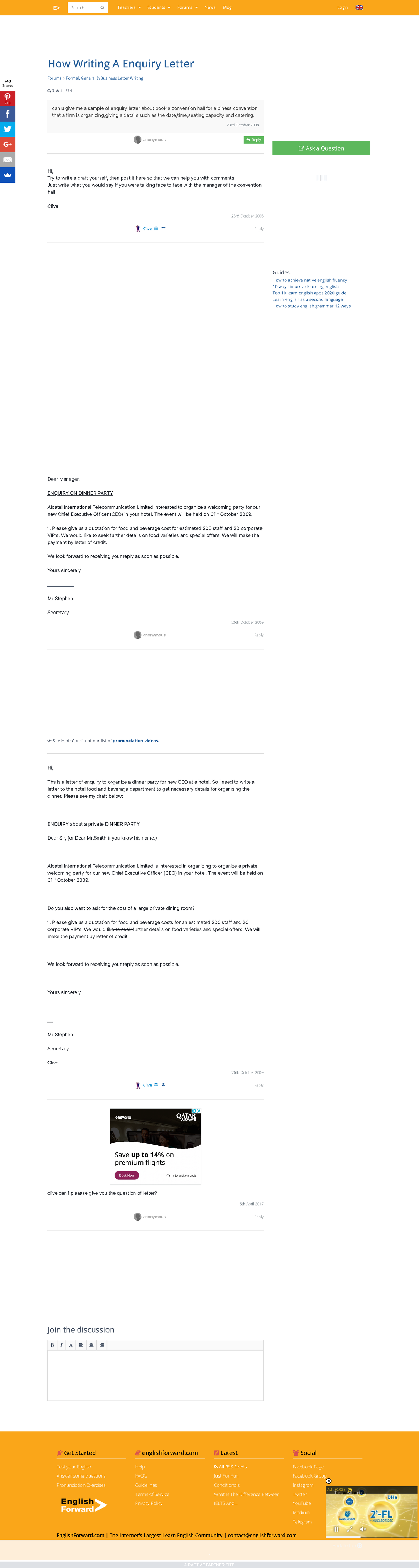The image appears to be a screenshot from a digital device, possibly a smartphone or computer. At the top of the screen, there is a long, slender, yellowish-orange header bar featuring clickable areas, including a search bar. Below this header, the content is displayed in a blueprint format. The main heading indicates "How to Write an Inquiry About a Letter," followed by small, less readable text. Two green clickable buttons with white text are prominently positioned beneath the heading.

On the left side of the screen, there is a vertical toolbar with social media icons, including Pinterest, Facebook ('F'), Twitter (bird), Google Plus ('G+'), and a couple more icons arranged vertically. The middle section of the screen is segmented by faint gray lines that divide various content areas. These sections contain text in very small print.

At the bottom of the image, there is an advertisement. The ad features a rectangle that is black at the top and white at the bottom, displaying the text "Save up to 14% on Premium Flights." Positioned below this message is a yellow rectangle, likely serving as a call-to-action button or an important highlight.

The overall layout of the screen is organized but cluttered, with the varying text sizes and colors drawing attention to specific areas while maintaining an integrated design.